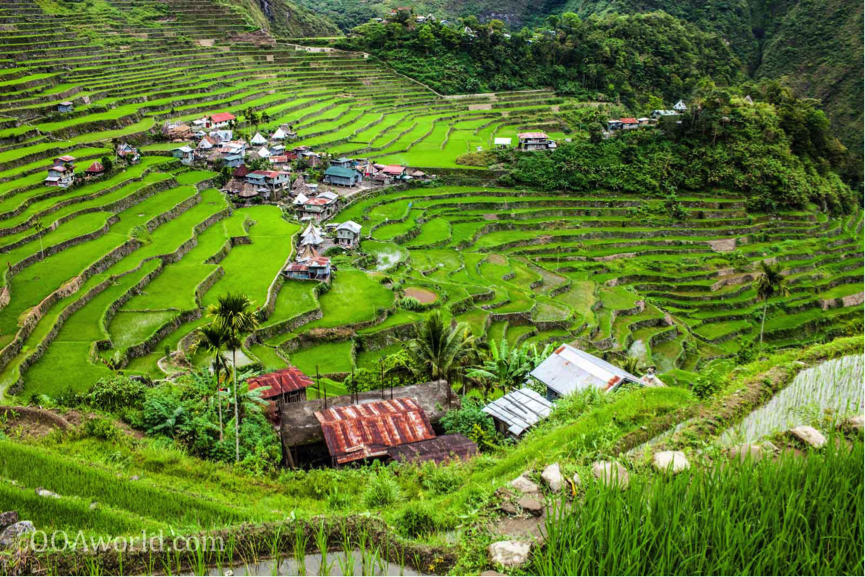The photo depicts an outdoor daytime scene featuring a layered, terraced landscape reminiscent of steps. A partly obscured website, showing as "aworld.com," is located in the lower left-hand corner. The setting includes a mix of farmland and residential structures. In the foreground, a cluster of red, brown, and white buildings is surrounded by numerous palm trees. Scattered throughout the image are various houses that stretch left and right and ascend a hillside on the right. The ground is lush with greenery, including dark green leafy trees, tall grass, bushes, and walkable paths. The background features cliffs or a mountainside, reinforcing the image's natural and varied terrain. The overall atmosphere of the scene is vibrant and detailed, capturing both the unique architecture and the abundant vegetation.